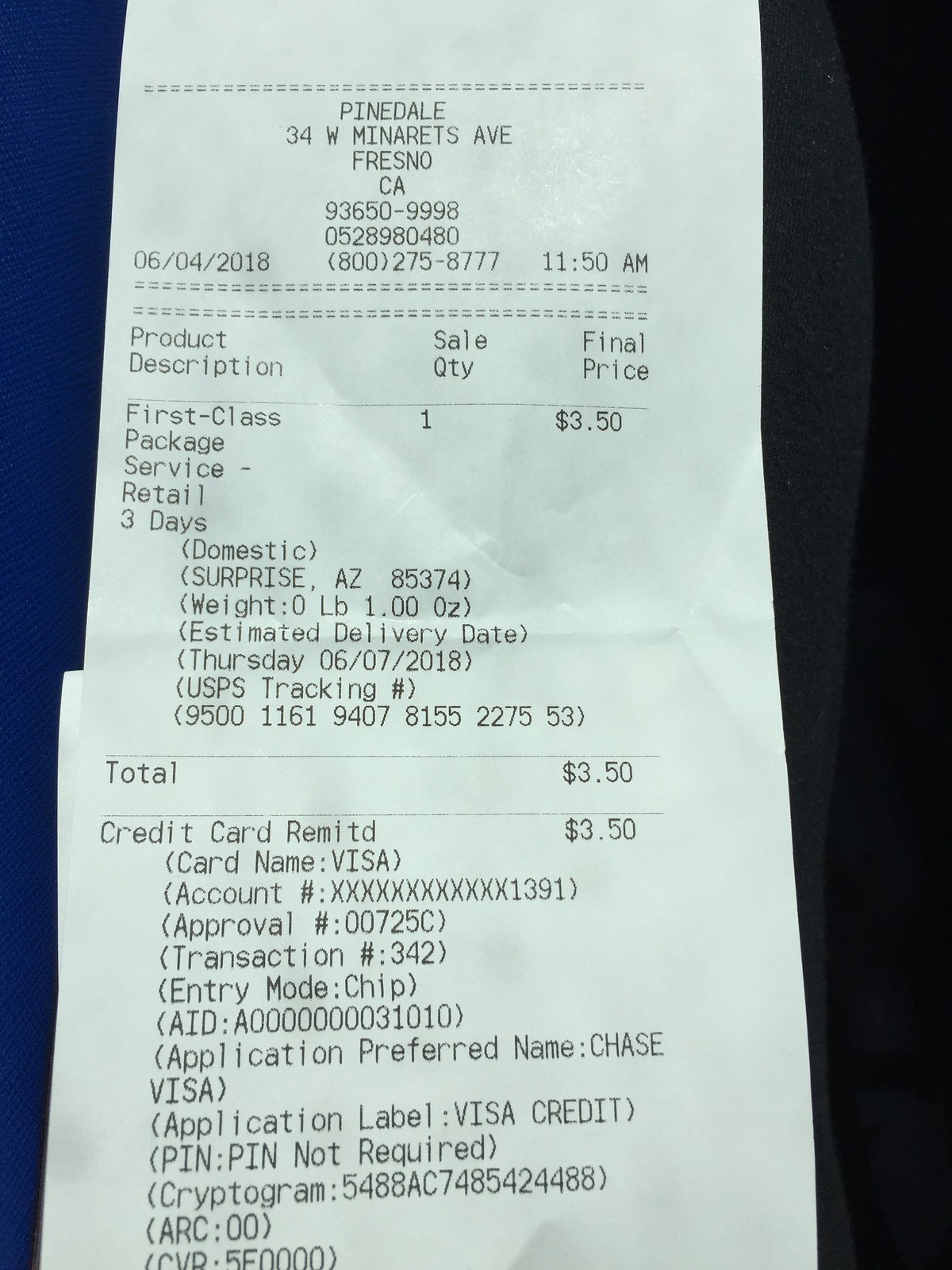This image depicts a detailed view of a receipt from a postal transaction at Pinedale, located at 34 W Minaretts Avenue, Fresno, CA 93650-9998. At the top, the receipt features the store information, followed by a transaction ID: 0528980480. On the left side, the date of the transaction is noted as 06/04/2018, with the time recorded at 11:50 a.m. To the right of the date, the contact number is listed as (800) 275-8777.

The middle section categorizes the purchase under "Product Sale" and describes the columns for "Description," "Quantity," and "Price." The first line item indicates a "First Class Package Service - Retail" dispatched domestically to Arizona, ZIP code 85374. The package weighs exactly 1.00 ounces, with an estimated delivery date of Thursday, 06/07/2018. The USPS tracking number associated with this shipment is 9500 1161 9407 8155 2275.

At the bottom of the receipt, the total transaction amount is noted to be $3.50, which was paid using a Visa credit card. The card details show "XXXX XXXX XXXX 1391" with an approval number of "00725C" and a transaction number of "342." The payment utilized chip entry mode, and other verification details include application data and cryptogram information. Due to the image cut-off, additional payment details and the receipt footer are truncated.

This document serves as a comprehensive record of an individual sending a package via first-class mail, complete with transaction and payment specifics.